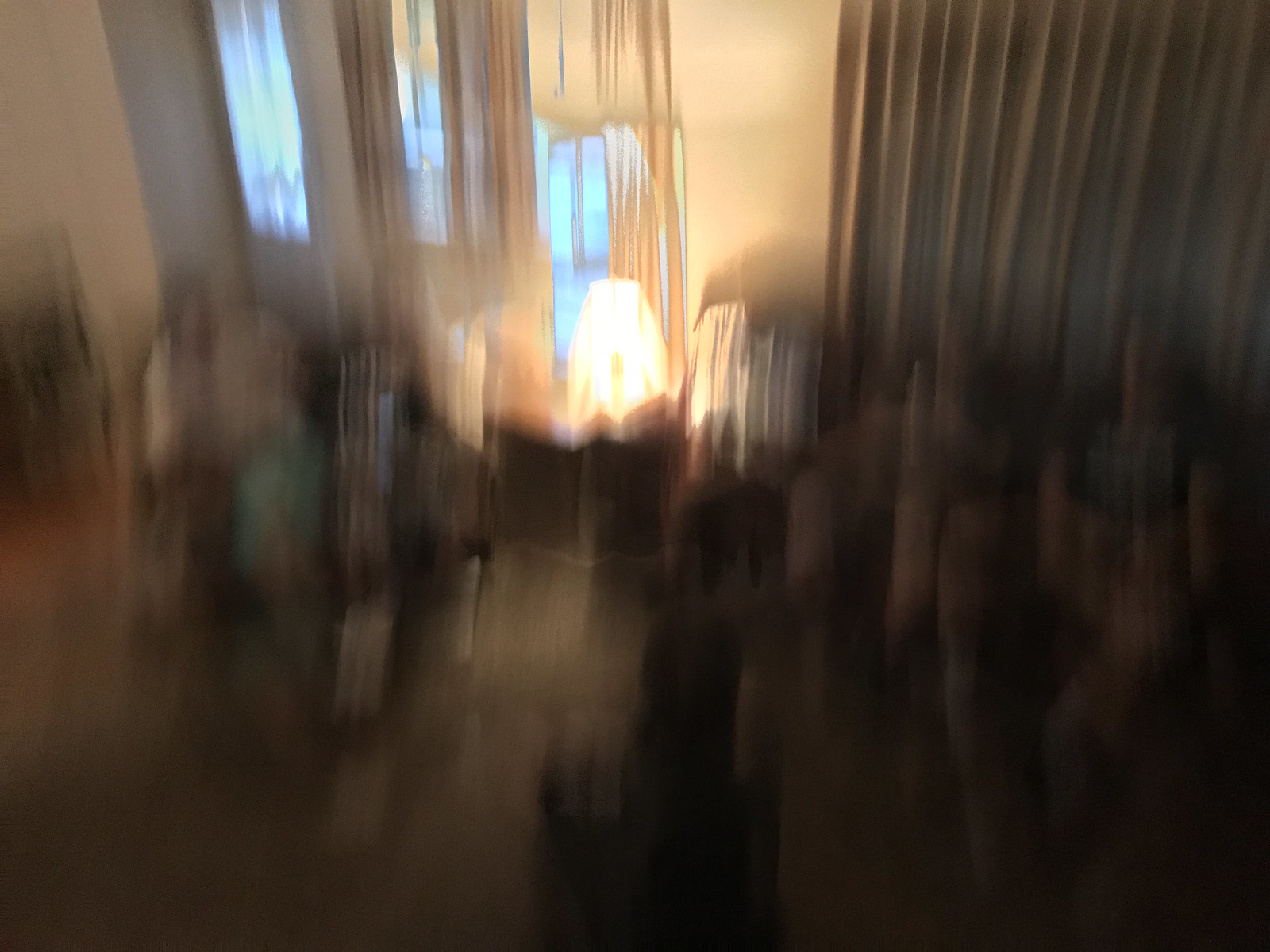This image is a photograph of a living room captured with significant motion blur, making details difficult to discern. On the left side, there’s a white wall with a light blue drape adjacent to it, partially covering a window with white sheers. This pattern of blue drapes and white sheers continues intermittently across the window that stretches toward the right. Sunlight filters through the curtains, adding to the blur effect. A brown carpet covers the floor at the bottom of the image. Toward the right, there is a couch where three people appear to be seated, two of whom are in front of the blue curtain, all dressed in shorts and t-shirts. A person in white is seated on a lounge chair to the left of the couch, next to a table with a lamp on it. A gray curtain hangs behind the couch, and there’s a door or window with glass panes emitting blue light in the upper right corner. The overall image is heavily distorted, suggesting it was taken with a low-quality camera in motion.